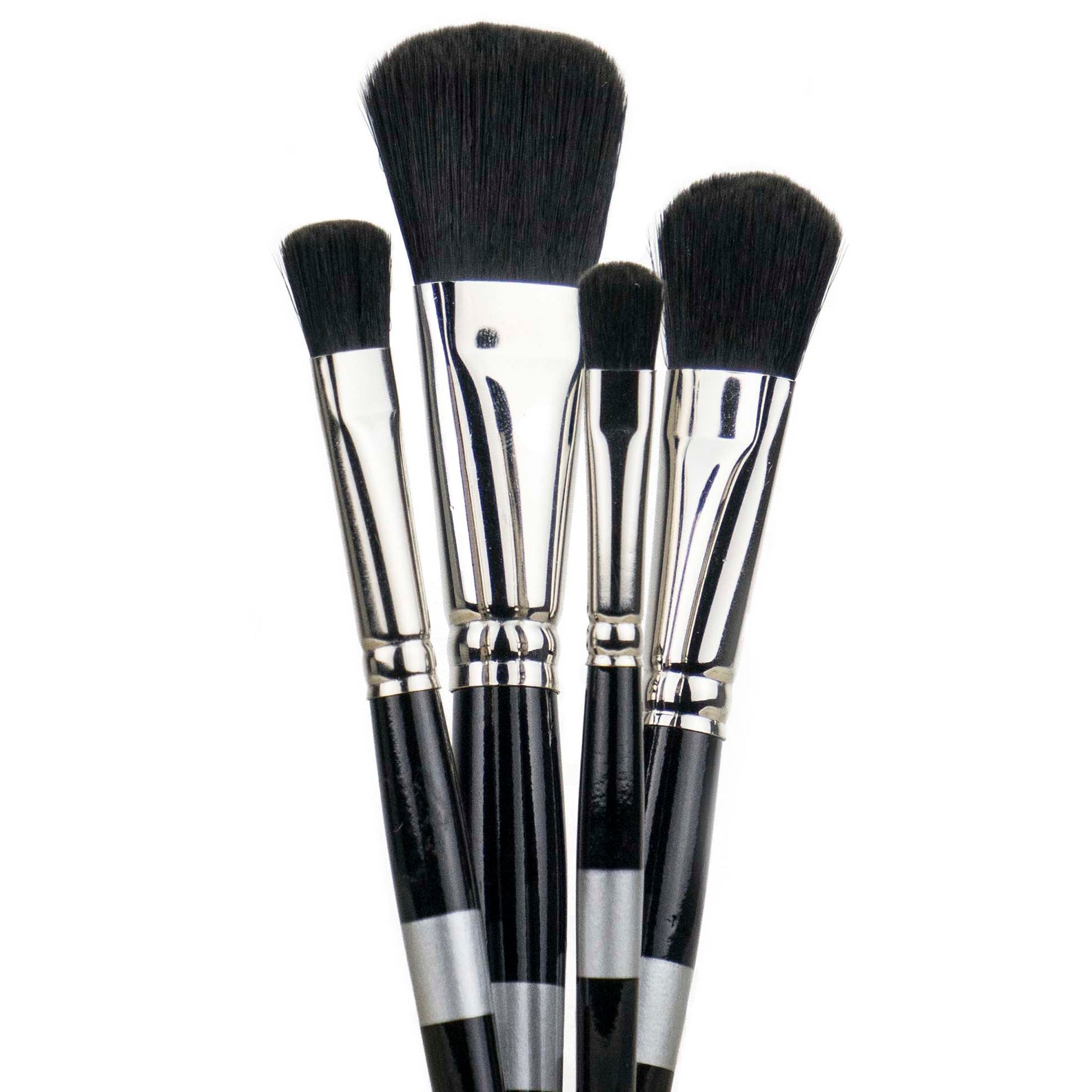This vertical, portrait-oriented image features a close-up of four makeup brushes set against a plain white background. The brushes' handles are cut off mid-length, allowing focus on their upper portions. Each brush showcases soft, black bristles that vary in size, with the largest brush centrally positioned and noticeably taller and wider, roughly five inches in height and an inch across at its broadest point. The smallest brush lies to the right, approximately four inches high and half an inch wide. All brushes feature shiny, silver metal ferrules that crisply secure the bristles, and two crimped areas that attach to the black wooden handles adorned with small silver bands lower down. The reflective silver parts emphasize the brushes' sleek, professional appearance, suggesting suitability for precise and effective makeup application.